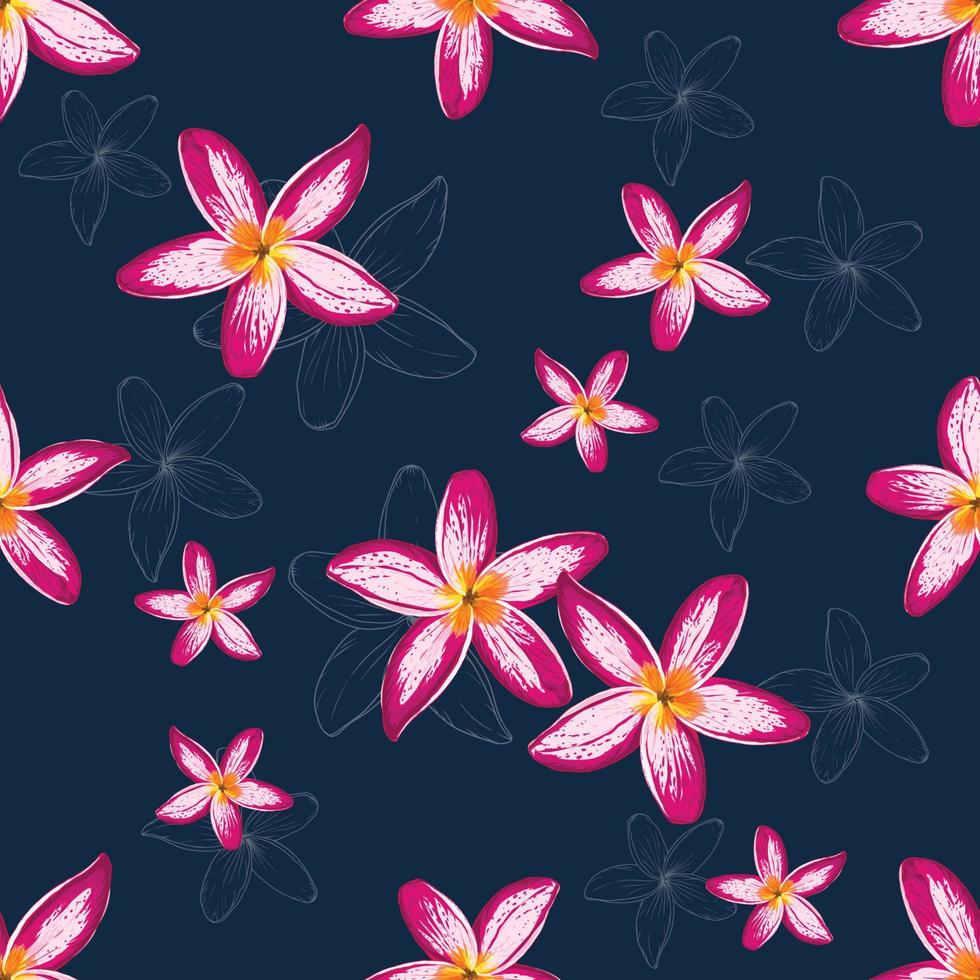This intricate piece of art showcases a striking floral pattern set against a deep navy blue background. The flowers, reminiscent of those one might find in the tropical settings of Hawaii or Florida, are vibrant with vivid hues of purple, pink, and red, accented by orange-yellow interior petals. Each flower, featured in various sizes, has five delicate petals adorned with subtle sprays of polka dots, adding texture and structure. The centers of these colorful blossoms are black. Interspersed among these vivid flowers are white, thinly sketched outlines of similar floral shapes, creating a harmonious balance between the colored and silhouetted elements. This combination of cheerful, brightly colored flowers and the contrasting dark background gives the entire piece a dynamic and uplifting feel.